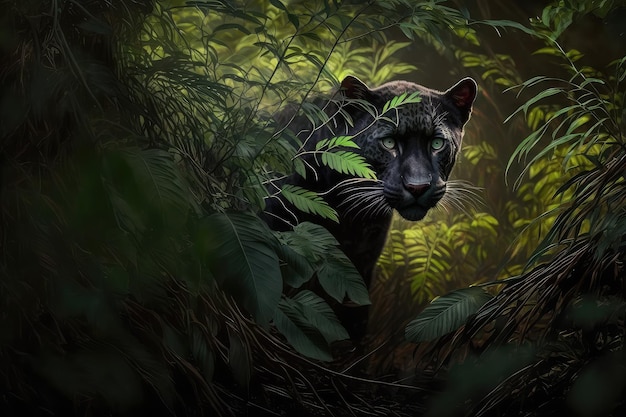In the dense, verdant jungle, a black panther emerges from the underbrush, its sleek, shadowy form partially obscured by the surrounding foliage. The foliage frames the panther, with a mixture of dark green leaves in the foreground transitioning to a lighter green further back. A subtle light source illuminates the central area, casting a glow that highlights the panther's face and piercing, lime-green eyes. The panther's spotted pattern is faintly discernible amidst its dark fur, and its white whiskers stand out sharply. Its head and upper body are visible through a small opening in the foliage, giving the impression that it is low to the ground, watching intently with a focused gaze. The scene evokes the mystique of a jungle, similar to imagery from the Jungle Book, with the leaves and branches largely obscuring the panther, except for this brief, luminous encounter.